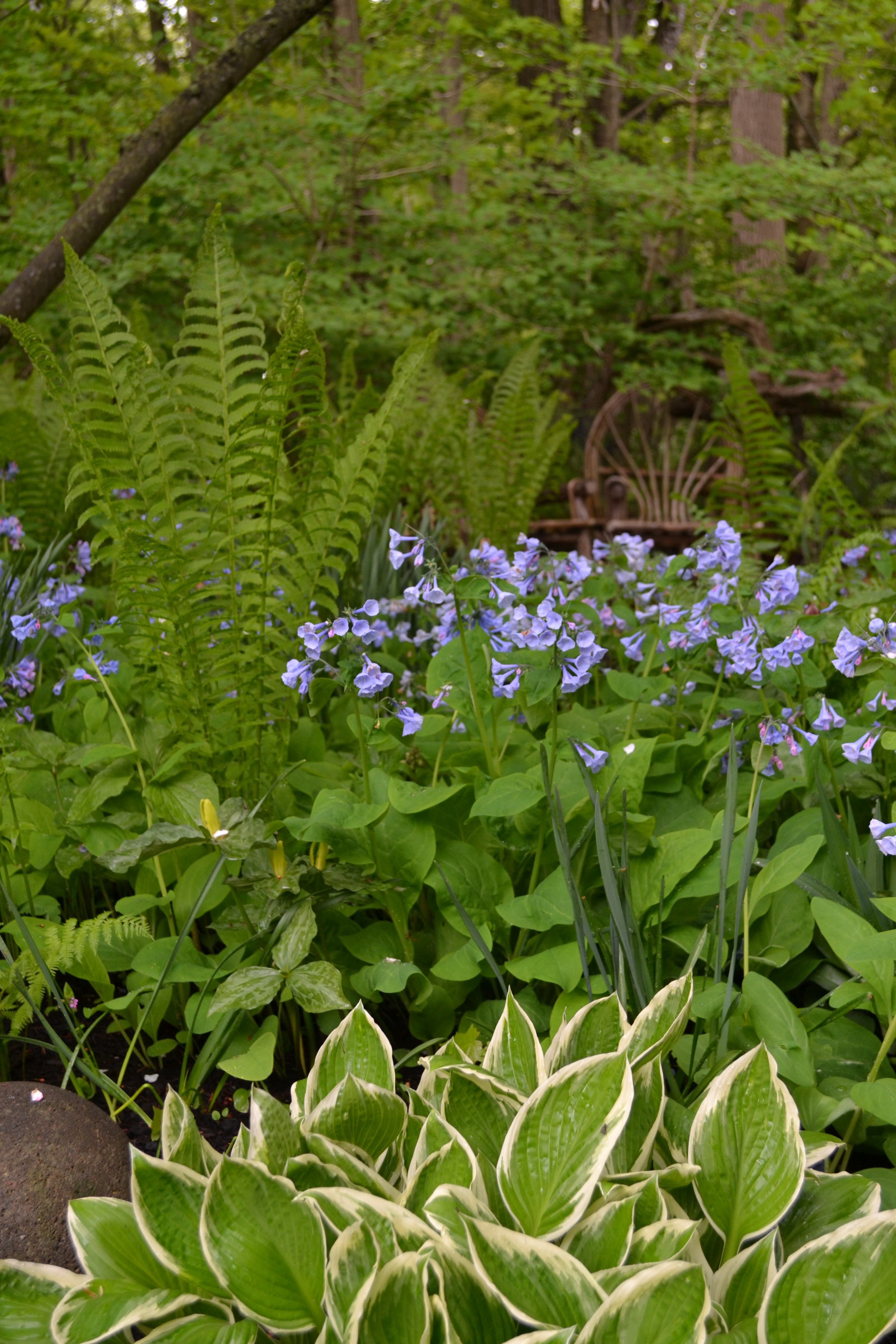In the image, we observe a lush garden characterized by a mix of various plants and features. Dominating the foreground are large hosta leaves, which are green with distinctive white edges, lending them a vibrant and healthy appearance. Nearby, a modest rock complements the natural setting. Clustered prominently in the center of the scene, delicate, bugle-shaped purple flowers, likely bluebells, bloom in groups of five to seven, adding a splash of color. Interspersed among these are elegant ferns with their fronds extending gracefully. On the left, tall fronds extend from a thin stem, creating a visually intriguing silhouette. Enhancing the garden's tranquil ambiance, a wicker or wooden chair is nestled amidst the greenery, providing a serene spot for rest and reflection. Providing shade and structure to the garden, a thick tree limb stretches diagonally across the top left corner of the image, while the background is framed by an array of trees. This detailed composition creates a peaceful and inviting garden scene.